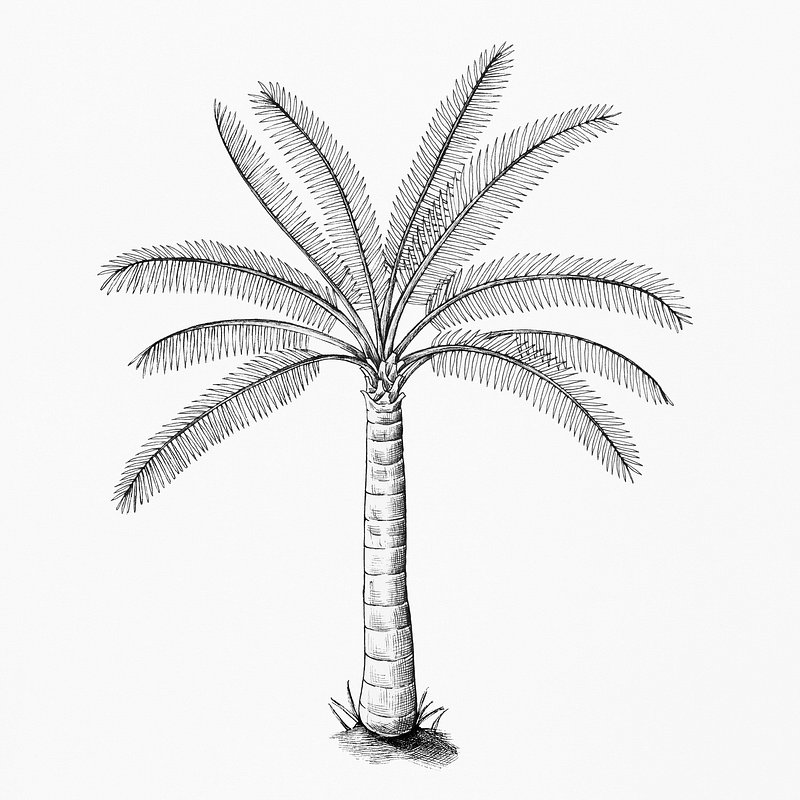This is a detailed black ink illustration of a palm tree standing upright against an almost white background that has a slight gray tinge. The tree has a straight trunk adorned with layered and shaded lines, leading up to where the ten fronds radiate from a single point at the top. These long, fanned fronds, seeming somewhat under the influence of normal gravity, point upwards and lack the typical droop. At the base, there are a few blades of grass sprouting around and some cross-hatching representing a small patch of ground, reminiscent of sand. We are viewing the tree head-on with a clearly detailed trunk and fronds but without any surrounding elements except the simple grass tufts and minimal ground shading. The overall style of the drawing is a stark, minimalist line sketch, emphasizing the simplicity and elegance of the palm tree.